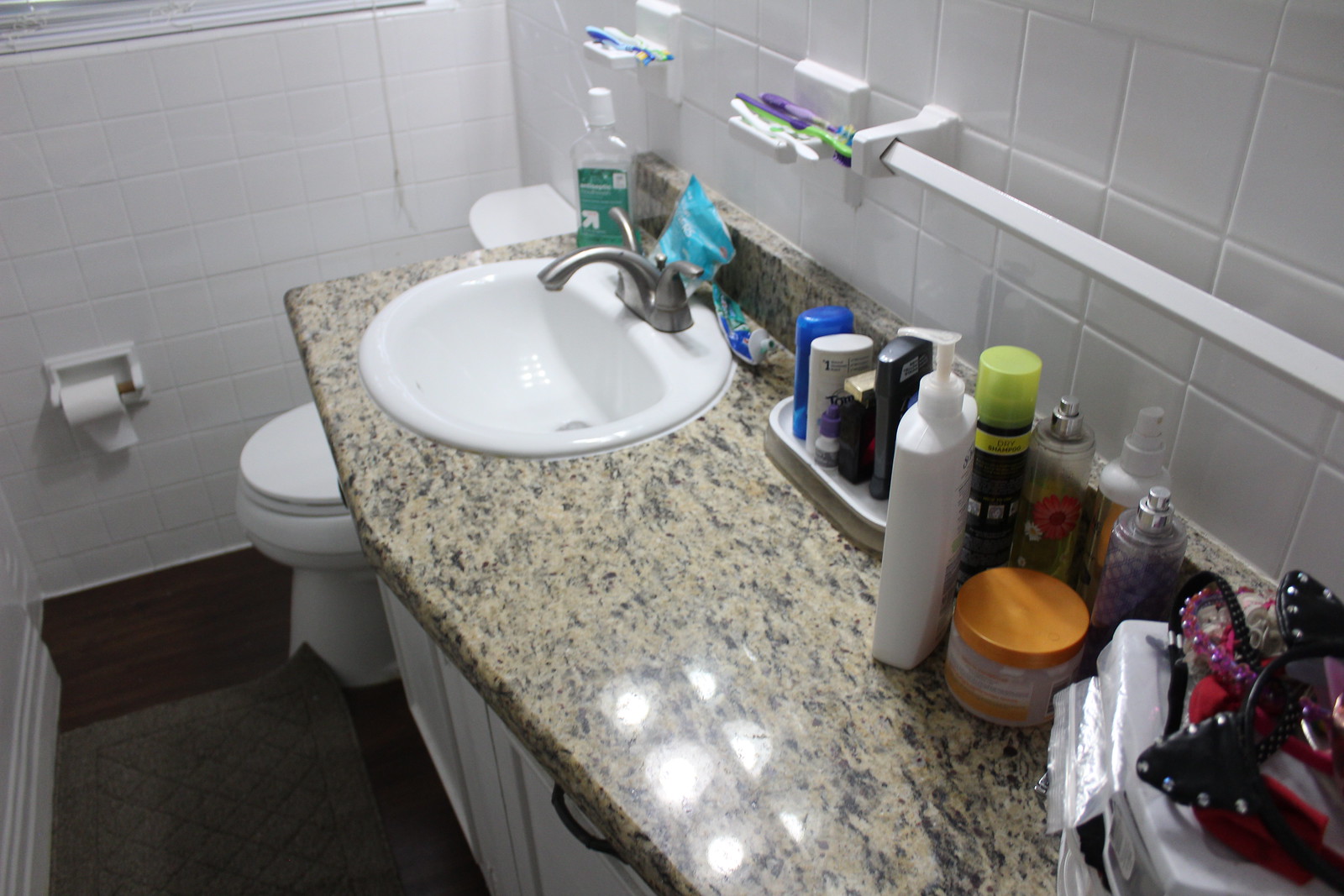Here is a detailed caption for the image:

The photograph depicts a meticulously organized bathroom featuring a gray and tan marble countertop. Positioned to the left is a sleek porcelain sink with a modern stainless steel faucet and dual handles for hot and cold water control. The expansive right side of the countertop is cluttered with an array of bathroom essentials, including various bottles of lotion, soap, hair sprays, deodorants, makeup remover, and perfumes, indicative of a well-stocked personal hygiene area. On the far left, a bottle of mouthwash with a prominent green label stands out.

Beyond the countertop lies a pristine porcelain toilet with its lid closed, accompanied by a toilet paper dispenser affixed to the wall, stocked with a roll of toilet paper. The bathroom walls are adorned with polished white tiles, maintaining a clean and bright atmosphere. Above the sink, two racks hold multiple toothbrushes, while a white towel rack is mounted on the far right, noticeably devoid of any towels. The overall image reflects a blend of functionality and cleanliness in the bathroom's design.